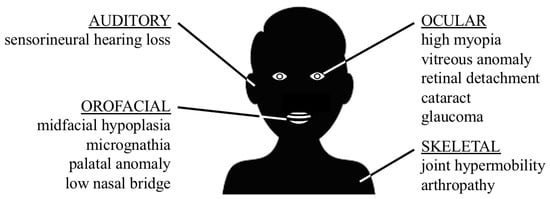This image is a black and white diagram, resembling a textbook or slide presentation. At the center is a black silhouette of a child with only white eyes and a slightly open white mouth. The diagram is labeled with text boxes highlighting various medical conditions associated with different parts of the body. 

In the top left, labeled "AUDITORY," with an arrow pointing to the ear, it describes "Sensorineural Hearing Loss."

Below that, labeled "OROFACIAL," with an arrow pointing to the mouth, it lists "Midfacial Hypoplasia," "Micrognathia," "Palatal Anomaly," and "Low Nasal Bridge."

In the top right, labeled "OCULAR," with an arrow pointing to the eye, it details "High Myopia," "Vitreous Anomaly," "Retinal Detachment," "Cataract," and "Glaucoma."

Finally, in the bottom right, labeled "SKELETAL," with an arrow pointing to the shoulder, it mentions "Joint Hypermobility" and "Arthropathy."

All these labels with corresponding arrows indicate symptoms or conditions affecting the ear, eye, mouth, and skeletal system, implying a complex health condition or syndrome affecting multiple body systems.